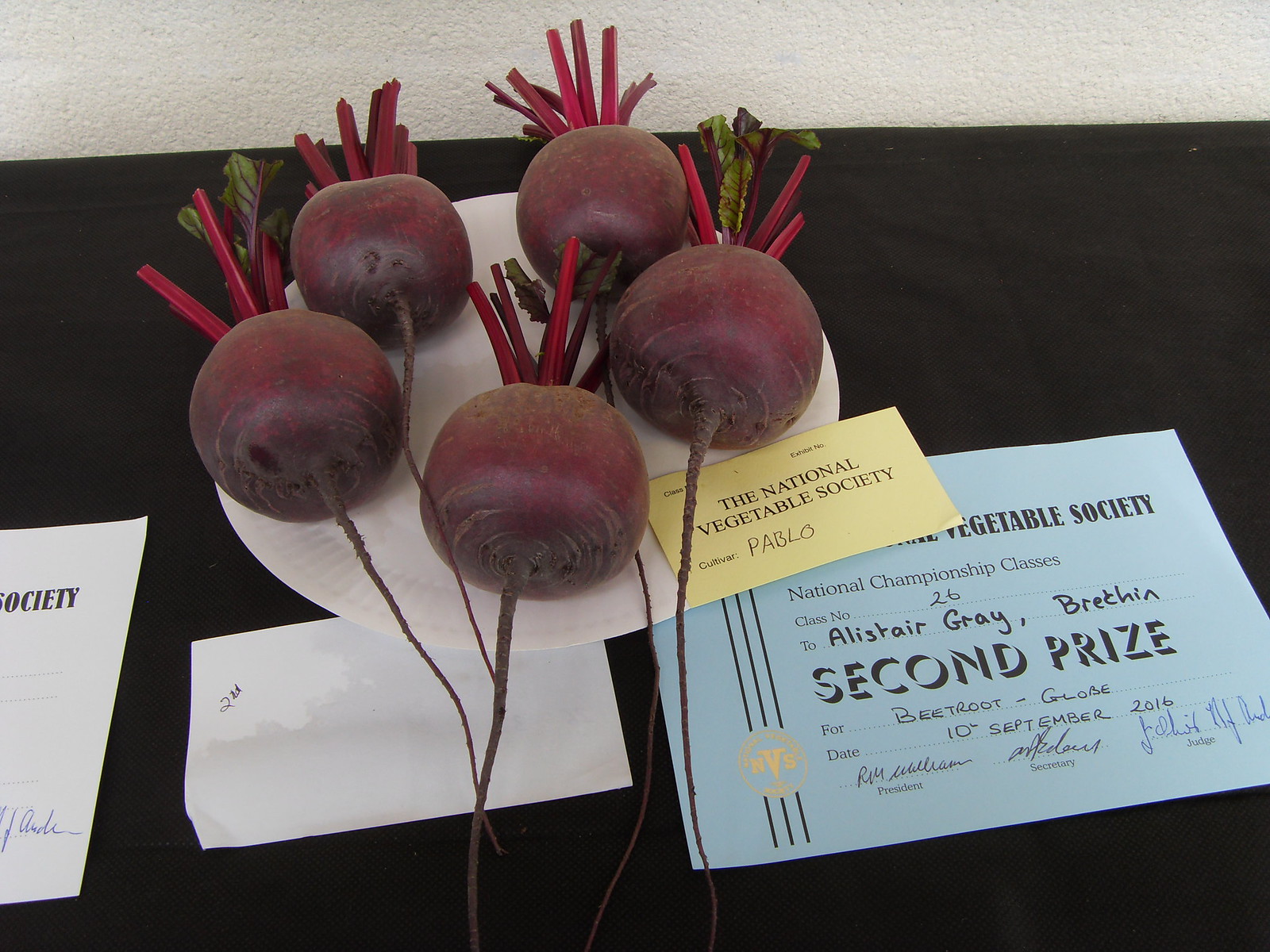The image showcases a close-up of a table covered with a black tablecloth, set against a white textured wall. At the center of the table is a white paper plate holding five meticulously cleaned beetroots, which have had their stems trimmed. Next to the plate, a yellow tag reads "National Vegetable Society" and identifies the cultivator as Pablo. Accompanying the display is a blue certificate adorned with a gold emblem, indicating that these beetroots won second prize in class number 26 for Beetroot Globe at the National Vegetable Society National Championship on September 10, 2016. The certificate is awarded to Alistair Gray from Brechin and bears the signatures of the President, Secretary, and Judge of the Society. Additional papers with the word "society" and a digitally altered note stating "second" further emphasize the achievement.